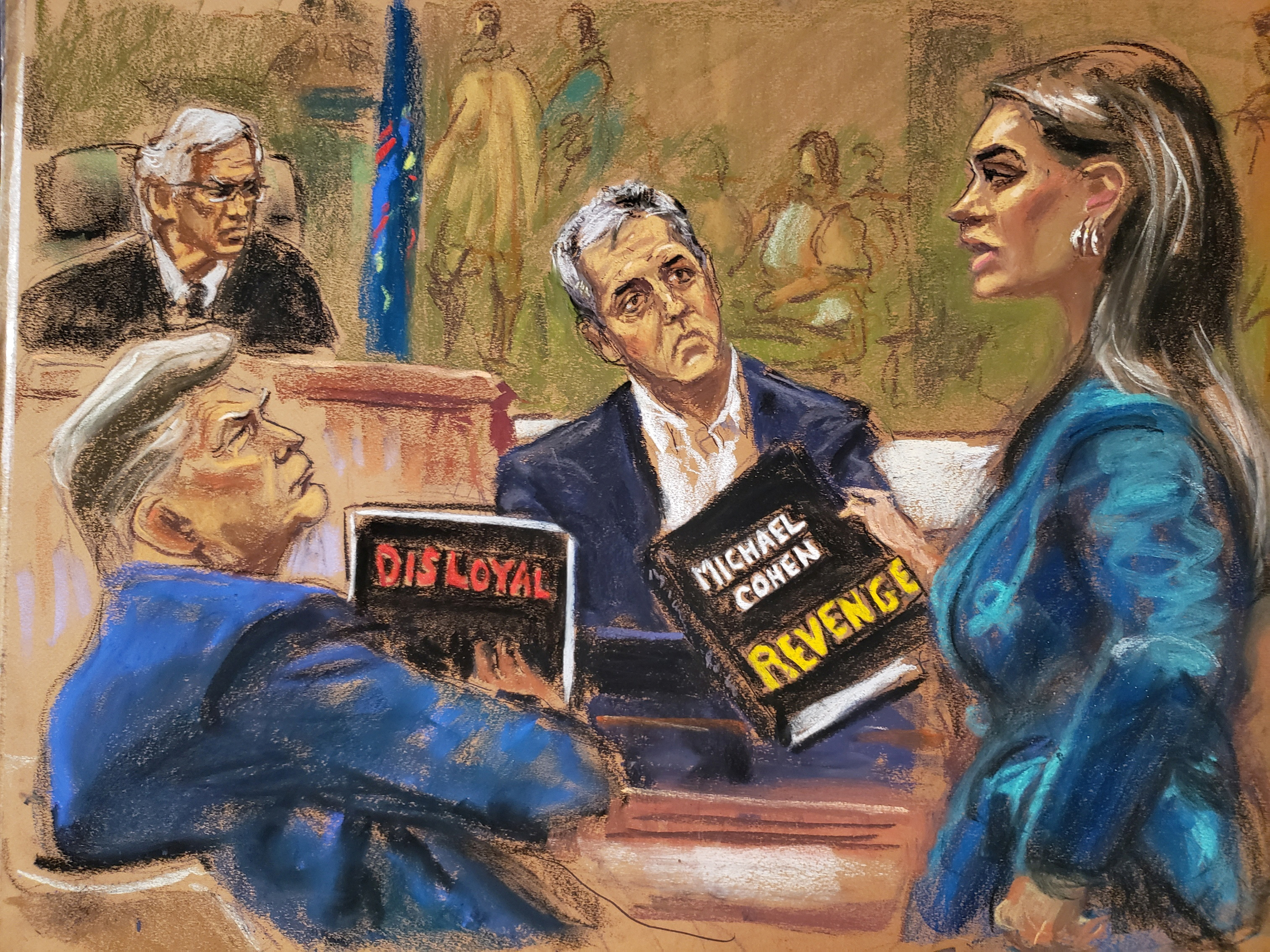The image is a detailed courtroom sketch featuring an artist's rendition of Donald J. Trump and other key figures in a trial-like setting. Donald Trump is prominent on the left side, facing a woman on the right, presumed to be his attorney, Alina Haba. Trump is holding a black book with "Disloyal" written in red text. Alina Haba, dressed in a blue blazer with makeup and brown hair, is holding a book titled "Michael Cohen Revenge" with white and yellow text. Standing beside Trump is another older man in a dark blue suit with grayish-white hair, seemingly observing Haba. Behind them, a judge with gray hair and glasses is seated at his bench, donning traditional black robes. A flag is positioned next to the judge. The background includes indistinct sketches of either a jury or audience members, adding depth to the courtroom scene. The features of the depicted individuals are slightly exaggerated, enhancing the artistic style of the sketch.